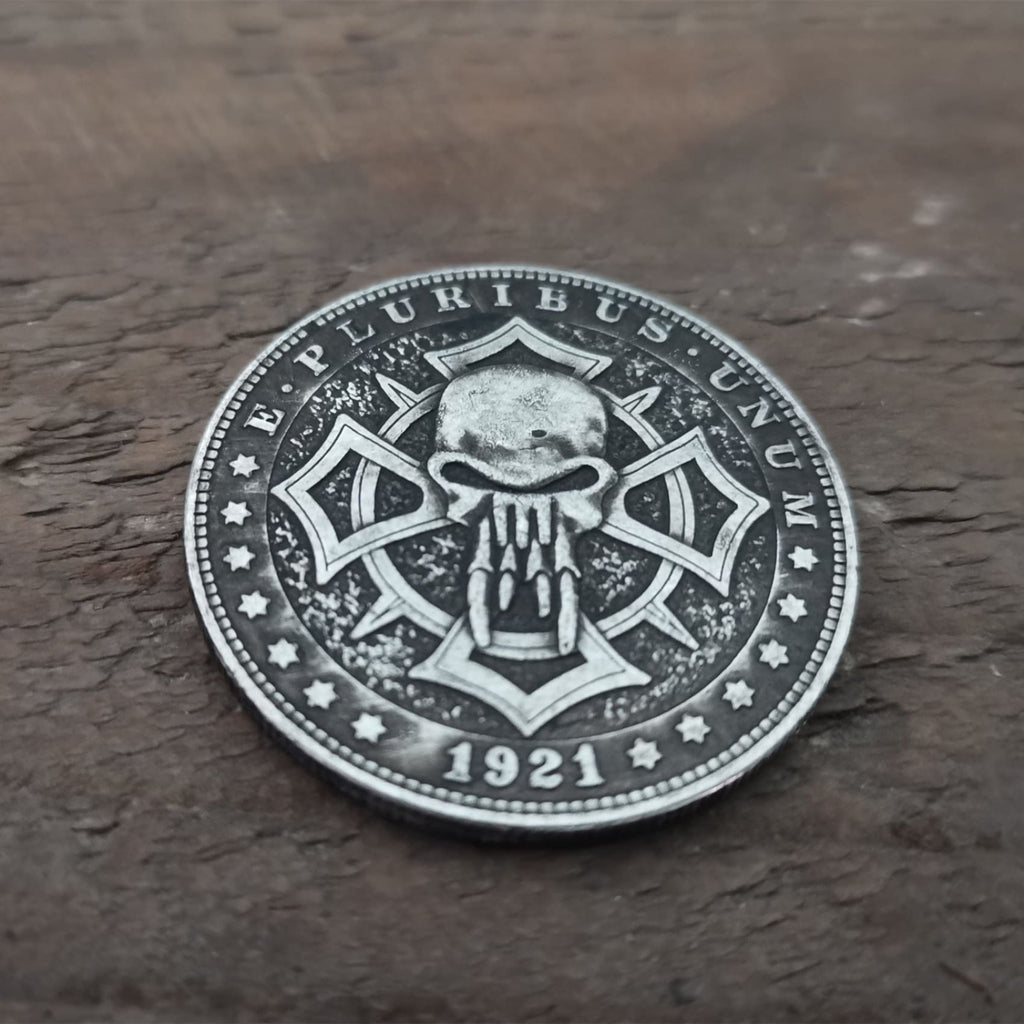This close-up image features a coin positioned against a dark brown, textured background that resembles ridged wood or layered rock. The coin is dark metal with a detailed silver outline, accented by a row of dots and a star border. At the top of the coin, the inscription "E Pluribus Unum" is displayed in silver letters on a black backdrop, and at the bottom, the date "1921" is similarly inscribed. Surrounding these inscriptions are several silver stars arranged along the coin's outer edge. The inner circle of the coin features silver flecks, and centrally, a striking design of a gray skull with four long vertical teeth dominates, flanked by diamond shapes extending from each side. This menacing skull design is further enhanced by a silver circle beneath it, perhaps suggesting a shield or protective armor. The composition highlights the fine details and craftsmanship of the coin against the contrasting textured background.